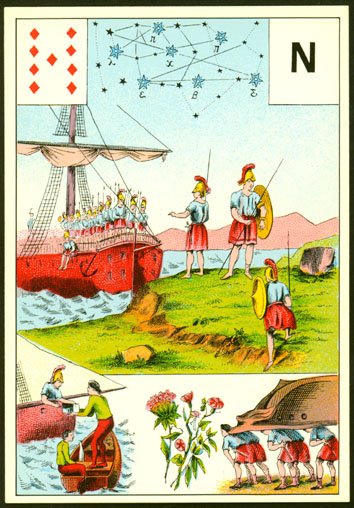This photograph depicts a detailed illustration on what appears to be a themed card. In the top right corner, the card is marked with the letter "N," and on the top left corner, there are nine red diamond shapes. In the center, stars interconnected are labeled with the letters "X," "E," and "B" in elegant cursive script.

The main visual element showcases an ancient Viking ship, richly painted in red, teeming with Viking warriors at its prow. The ship has its sail furled, indicating it is docked or preparing to dock. The scene is set against a backdrop of blue waters. 

To the right, three Viking warriors are depicted standing on a grassy shoreline. They are prepared for combat, holding round shields and long spears, creating a poised and dramatic scene.

Below the central image, another scene displays five Vikings bent over, seemingly engaged in lifting or carrying a wooden structure. The middle of this image is adorned with vibrant pink flowers, complete with green leaves and stems, adding a touch of nature to the stark Viking activities.

On the left side of the card, a smaller boat approaches the Viking ship. This boat carries individuals dressed in green shirts and red pants, distinctly different from the Viking warriors, indicating that they might be from a different group or community, possibly coming to trade or communicate.